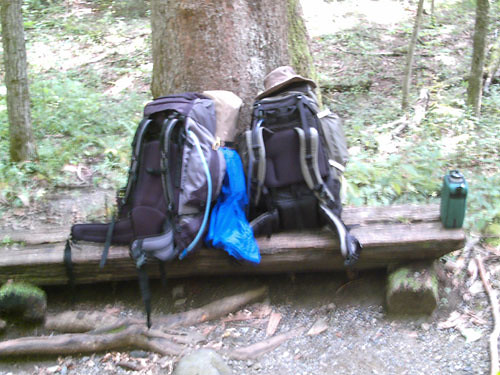This photograph captures two large, fully-packed hiking backpacks resting on a split-log bench in the midst of a wooded area. The bench, formed from a log split in half with the flat side up, is supported by two additional logs lying horizontally beneath it. Dominating the center of the scene is a thick tree trunk, surrounded by other trees, contributing to the forested backdrop. The ground is a mix of dark brown soil, patches of green grass, and scattered broken limbs and logs.

The backpacks, which are dark gray with lighter-colored straps and some blue and tan accents, sit atop the bench with their shoulder straps facing outward. The left backpack partially conceals a blue tarp near its base and has a tan covering around its upper section. The right backpack is topped with a light tan hiking hat. Positioned to the far right of the bench is a rectangular green canister, likely a water container. The photograph is slightly blurry, suggesting some motion occurred while the image was being captured. Overall, this scene portrays a tranquil outdoor setting with essential hiking gear ready for an adventure.